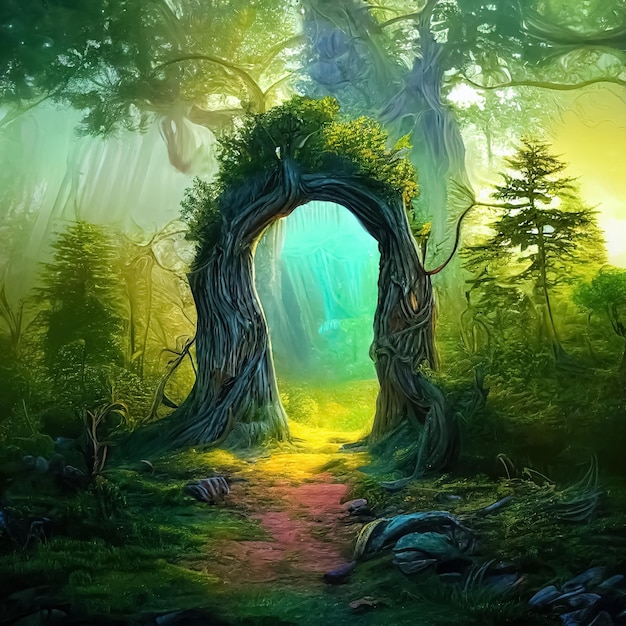This animated or illustrated artwork depicts a whimsical and fantastical forest teeming with life and vibrant colors. At the center of this scene is an archway woven from the roots and branches of ancient trees, forming a natural portal that radiates magic. Verdant greenery adorns the top of this arch, adding to its enchanting appeal, while a well-worn clay-colored path, dotted with boulders and roots, leads through it. The ground leading up to the portal is speckled with intriguing pink hues, which then transform into a mesmerizing yellow, ultimately giving way to a neon blue glow inside the portal itself. This glowing interior starkly contrasts with the lush, sun-dappled forest outside, where the sunlight cascades through the canopy, illuminating the vibrant green leaves and casting ethereal shadows. Surrounding the arch are smaller, scrubby pine trees, adding texture to the scene, and at the back stands a grand, gnarly tree with a burled trunk, adding to the surreal and mythological atmosphere. The sun, setting in the background, bathes the forest in a warm, golden light, heightening the sense of magic and wonder in this mythical woodland.